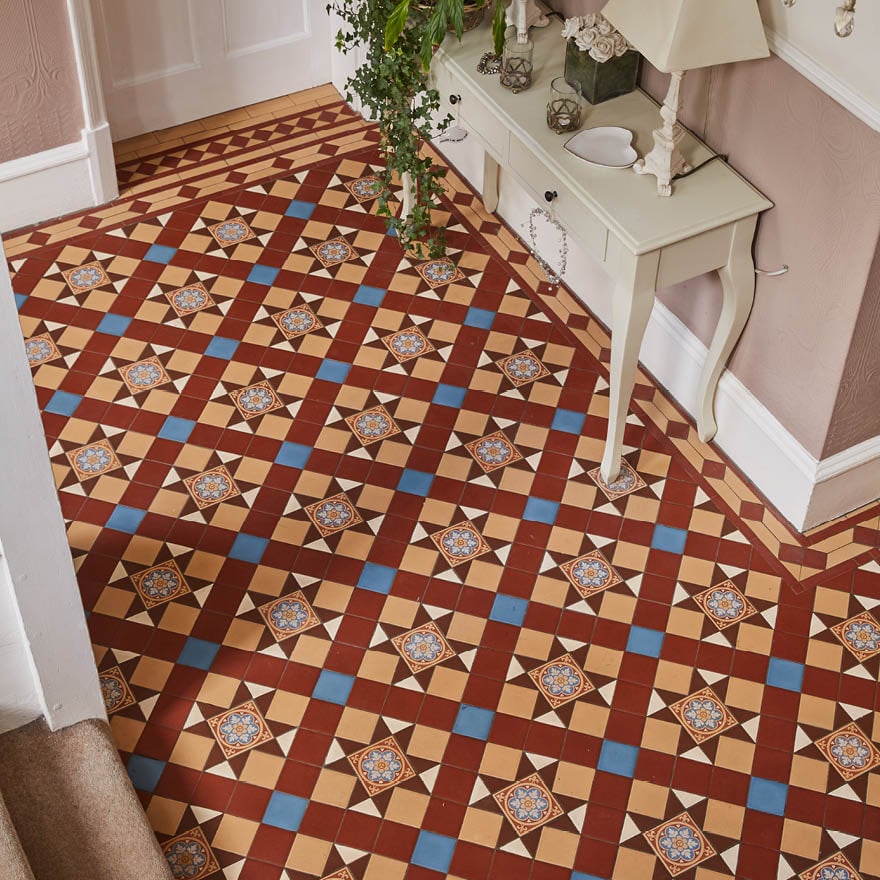The image depicts an intricately designed entryway in a home, potentially influenced by architectural styles from regions such as Mexico, South America, India, or Pakistan. The floor captures immediate attention with its elaborate geometric tiling, featuring a vibrant diamond pattern using colors like blue, rust, tan, and deep red. Central to the design is a starburst motif crafted from triangular cream and dark brown tiles, surrounding a delicately painted porcelain tile that resembles the Star of David.

Adjacent to the floor is a simple yet elegant setup against a beige wall with white baseboards and trims. A white wooden side table sits beneath a white-framed doorway, holding various decorative items. On the table, there's a small lamp with an ornate metal base, a gray vase filled with white roses, a heart-shaped white dish trimmed with gold, and a potted plant with green tendrils cascading downwards. The scene also includes two small glass candle holders. Visible at the bottom left corner are the initial steps of a staircase, covered in beige carpet. Together, these elements create a welcoming and aesthetically pleasing entryway.